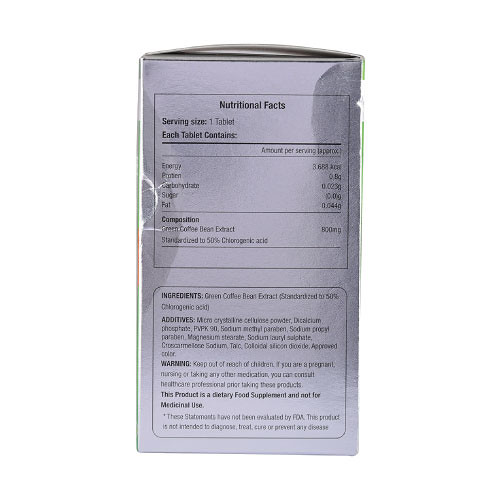This photograph captures the side label on a rectangular, white cardboard box containing a food supplement. The box appears slightly wrinkled, indicating it may have been squeezed or crushed. The detailed nutritional facts specify that each serving size is one tablet, with each tablet providing energy, protein, carbohydrates, sugar, and fat. The main ingredient is prominently listed as green coffee bean extract, totaling 800 mg per tablet. Additionally, there is a clear warning advising to keep the product out of reach of children, alongside other important ingredient and product information.